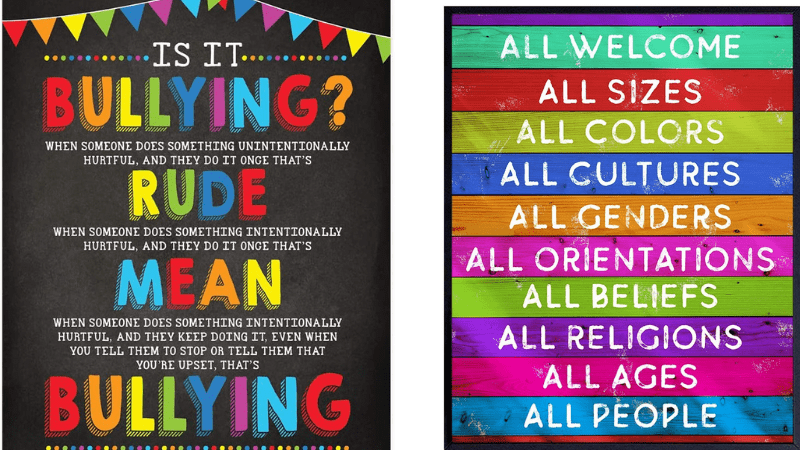In the image, there are two brightly colored classroom posters side by side, both promoting inclusive and anti-bullying messages. The poster on the left has a black background with vibrant, multicolored text and pennants in hues of red, orange, green, blue, and purple decorating the top. It poses the question, "Is it bullying?" in rainbow-colored letters with an orange question mark. The subsequent white text defines different harmful behaviors: rude (unintentionally hurtful actions done once), mean (intentionally hurtful actions done once), and bullying (intentionally hurtful actions done repeatedly, even after being asked to stop or expressing upset). 

The poster on the right features staggered, colorful boards from top to bottom—each a different color (blue, red, yellow, green, orange, purple, pink)—with "All Welcome" statements listed in bold white text. It reads: "All sizes, all colors, all cultures, all genders, all orientations, all beliefs, all religions, all ages, all people," and is framed by a black border, emphasizing the inclusivity message. Both posters are designed to enhance a supportive, diverse, and respectful environment.